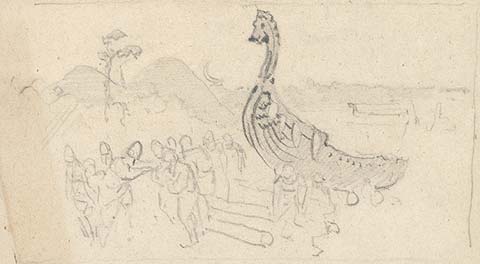This horizontally aligned, rectangular drawing, rendered in shades of gray, features a minimalist, hand-drawn scene on what appears to be a sheet of art paper. The solid gray background varies slightly in shade, with a darker gray on the far left. The central focus of the drawing is a large animal, likely a dinosaur with a tall neck and spikes running down its back, resembling a banana in shape. To the left of this creature are outlines of people, appearing to push against or interact with something indeterminate. These figures, along with the dinosaur, suggest a possible narrative moment.

In the distance, simple curved lines hint at hills, with tree-like squiggly lines extending upwards. The entire drawing is sketched with pencil, lacking intricate detail but providing a clear, evocative scene. The composition indicates an outdoor setting, despite the rough, impressionistic quality of the artwork. This piece captures a moment of interaction between humans and a large creature set against a faint, natural backdrop of hills and trees.